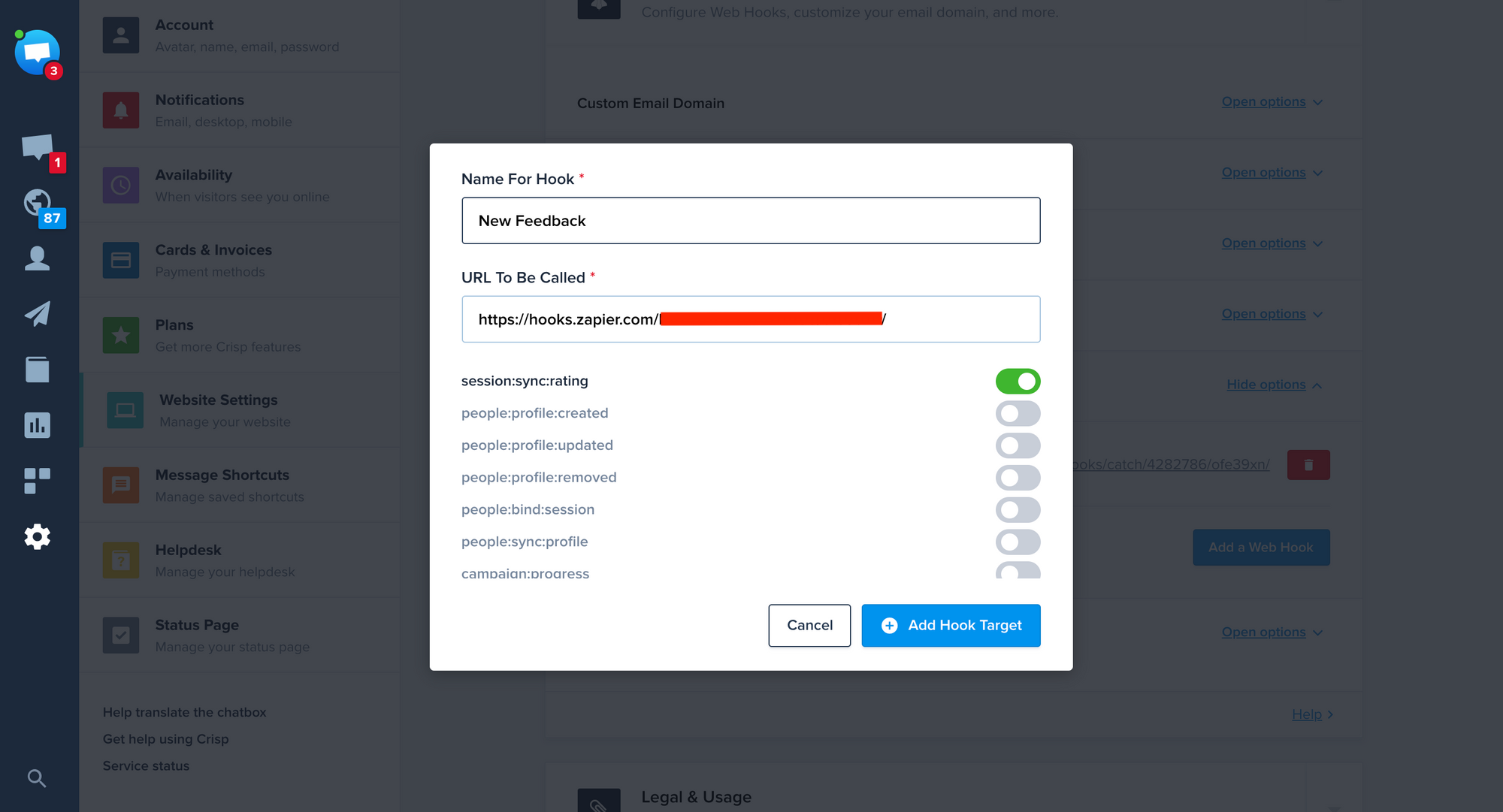This screenshot captures a website or application interface. On the left side, there is a dark blue sidebar featuring a variety of icons. At the top of the sidebar, a blue gradient circle displays a white chat box icon. A small green circle overlaps its upper left edge, while a larger red circle with a white numeral '3' encroaches on the lower right.

Beneath this section, with some spacing in between, a slightly tilted light blue chat box icon is accompanied by a smaller red rectangle on its lower right, showing a white numeral '1'. Following this, a series of blue icons are arranged vertically:

1. A globe icon with a blue rectangle on its lower right, displaying the white numerals '87'.
2. A profile picture icon.
3. A paper airplane icon.
4. A book icon.
5. An icon of a chart with dark blue bars.
6. An icon with three separated squares (two in the first row and one at the top of the second row).
7. A white cog icon.

At the bottom of the sidebar, after some additional spacing, there is a medium gray magnifying glass icon indicating a search function.

To the right, the main content area of the page is significantly darkened. Overlaying this darkened area is a white popup window. At the top left of the popup, dark gray text reads "Name for hook" followed by a red asterisk, indicating a required field. Below this text is a text entry box with a dark gray outline, containing the placeholder text "new feedback" in black.